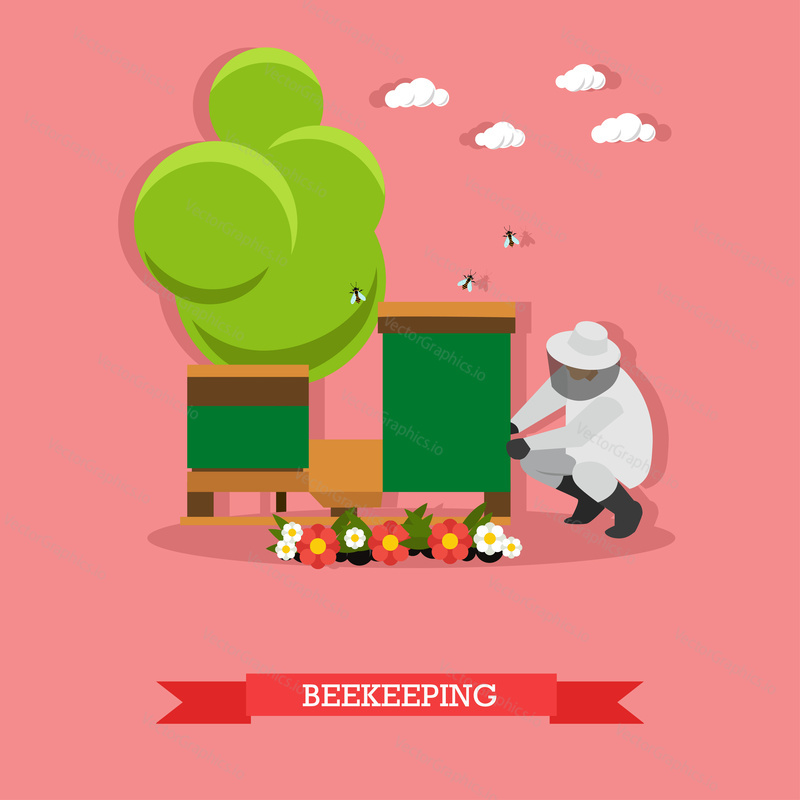The animated, or possibly computer-generated, image features a cartoon-like scene set against a vibrant pink background with scattered white clouds. In the foreground, a beekeeper dressed in a white suit is bent over, attending to the tallest of two bee houses, both having green, brown, and orange hues. Three bees are seen escaping the green section of the bee houses, flying upwards. To the right of the beekeeper, and behind the smaller bee house, stands a tree with dense, illustration-like green foliage made up of numerous circular shapes. At the base of the bee houses, there are daisies and other flowers in red and white. Adding detail to the scene, a banner at the bottom displays the word "Beekeeping" in white letters set against a red ribbon. The image is marked with a watermark from vectorgraphics.io, which is not clearly visible.